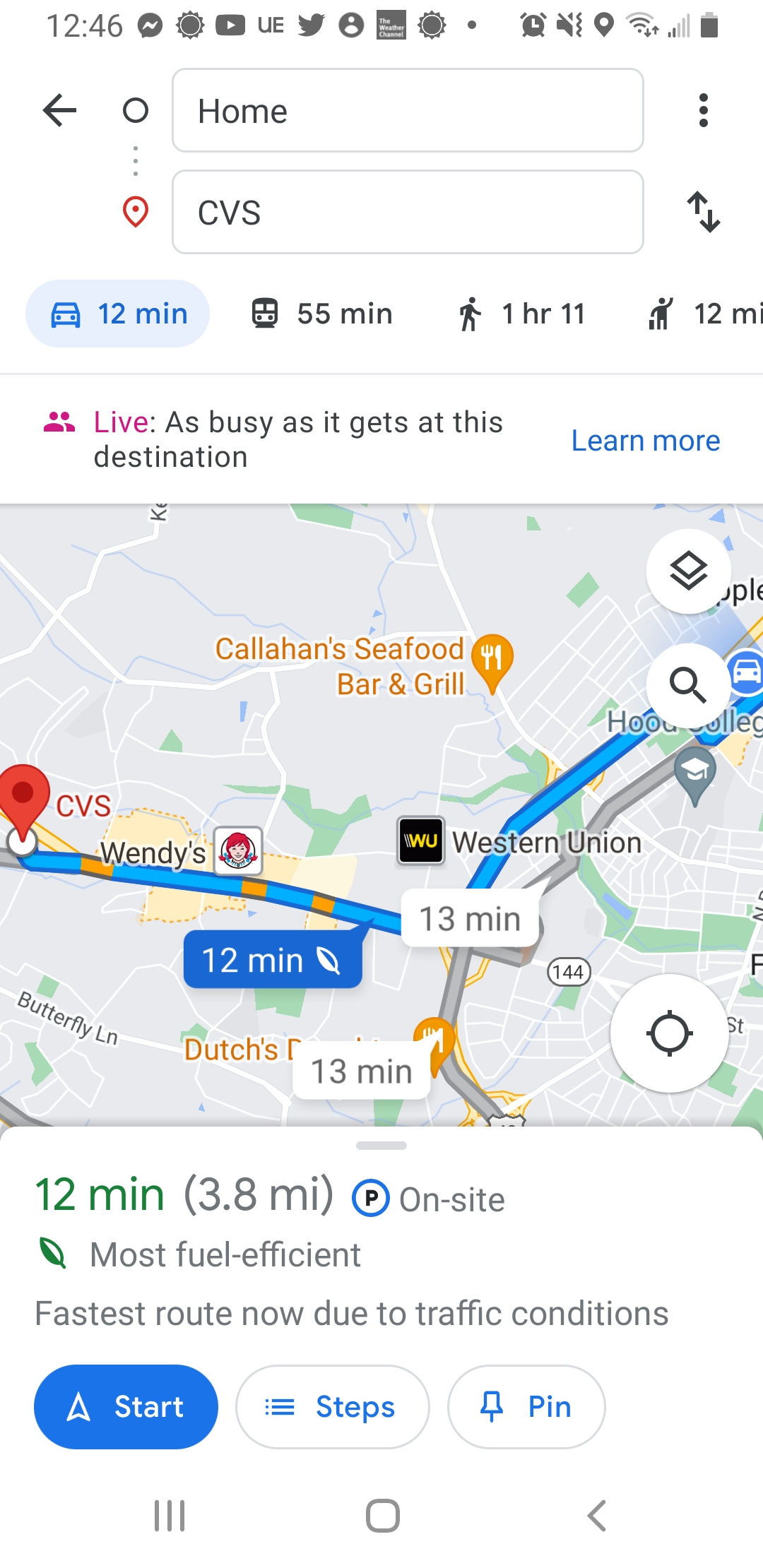This screenshot captures a user's cell phone display while navigating to a CVS pharmacy. The phone's status bar at the top displays various standard icons like signal strength, battery level, and time. The displayed application shows the user's current location as "Home" with CVS as their destination.

The navigation directions reveal multiple travel options: a 12-minute drive (covering 3.8 miles), a 55-minute bus ride, a 1 hour and 11-minute walk, and a 12-minute commute using another mode of transportation. The interface presents a detailed map highlighting significant landmarks and businesses along the route, such as Callahan's Seafood Bar, a Western Union, a Wendy's, and the CVS itself. Options to start the journey, view steps, and pin the destination are visible below the map. The image contains no human figures.